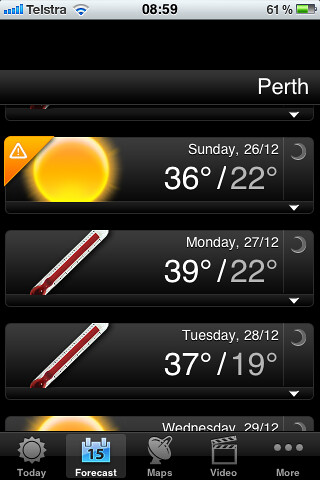This image is a detailed screenshot of a smartphone displaying a weather forecast for Perth. At the top of the screen, the time is shown as 8:59, with a status bar indicating a 61% battery charge, Wi-Fi connectivity with 2 out of 3 bars, and a full 5-bar connection to Telstra. The background transitions from a blue strip at the top to black. Below, the forecast begins with Sunday, 26-12, showing a high of 36°C with a bright sun icon and a low of 22°C with a small moon icon. Monday, 27-12, features a red thermometer icon with temperatures at 39°C high and 22°C low. Tuesday, 28-12, shows another red thermometer with a high of 37°C and low of 19°C. The top of the word "Wednesday" is visible at the bottom, accompanied by a sun icon. At the very bottom, there are icons labeled "Today," "Forecast," "Maps," "Video," and "More."